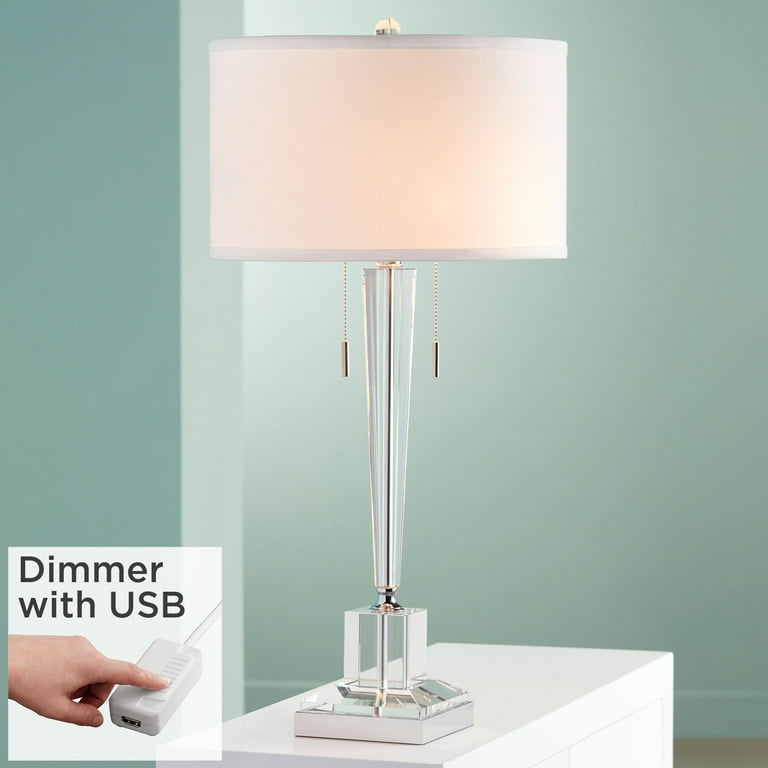This photograph is a detailed, well-styled product image intended for an advertisement or catalog. It features a tall table lamp with a sophisticated, clear glass base that forms a reverse triangle, resting on a pristine white table. The base integrates both solid and clear elements, adding a contemporary touch. The neck of the lamp also continues the clear aesthetic, resembling a cylindrical shape. The lamp is topped with a plain white linen lampshade, and a sleek, matching clear glass knob sits at its peak.

The lamp's functionality is highlighted by two metal pull chains, suggesting dual bulbs for adjustable lighting. In the background, indoor walls painted in varying shades of green and blue create a serene, aqua-toned ambiance. Additionally, there's an inset image at the lower corner of the photograph displaying a dimmer with a USB port, emphasizing the lamp's modern, multi-functional design. This inset includes an image of a hand using the USB dimmer, signifying easy control and added convenience for the user.